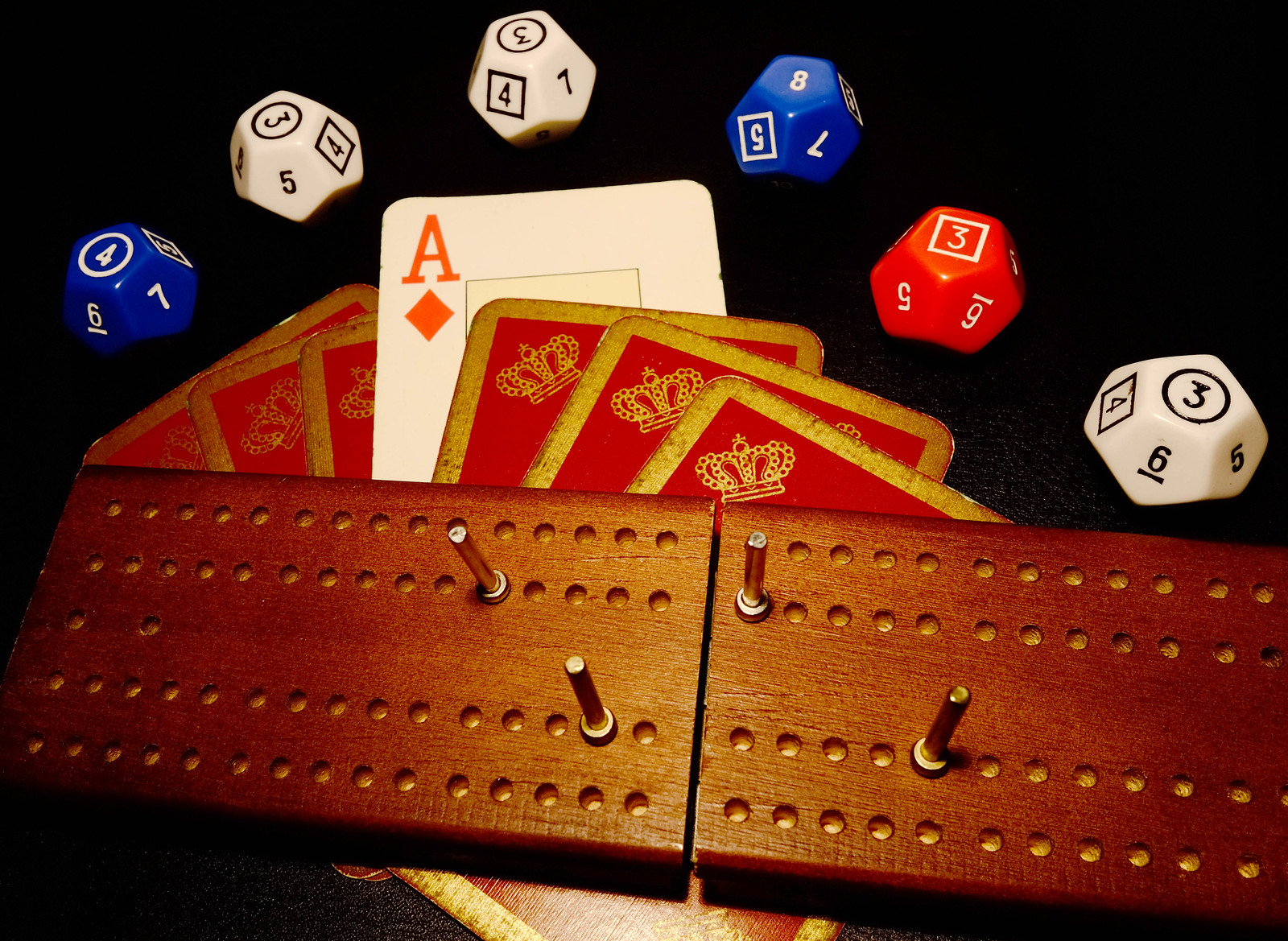Against a black background, the image showcases six nine-sided dice and an assortment of playing cards arranged in an intricate display. Starting from the left, the first die is blue, displaying the number four on its top face. Next to it, a white die features the number three. At the top center of the image, another white die prominently displays the number three. Moving right, a blue die shows the number eight, and below it, an orange die is marked with the number three inside a square. Completing the lineup, a white die features the number three encircled in a round border.

In front of the dice, seven playing cards are fanned out on the table. The cards are predominantly red with gold trim and feature a crown in the top left corner. The fanned arrangement highlights the ace of diamonds, prominently raised in the center. Overlapping the cards is a wooden board with a series of small holes organized in two rows at the top and two rows at the bottom. The board is punctuated by a silver peg positioned at the top and bottom of each row, contributing to the intricate and detailed composition of the scene.